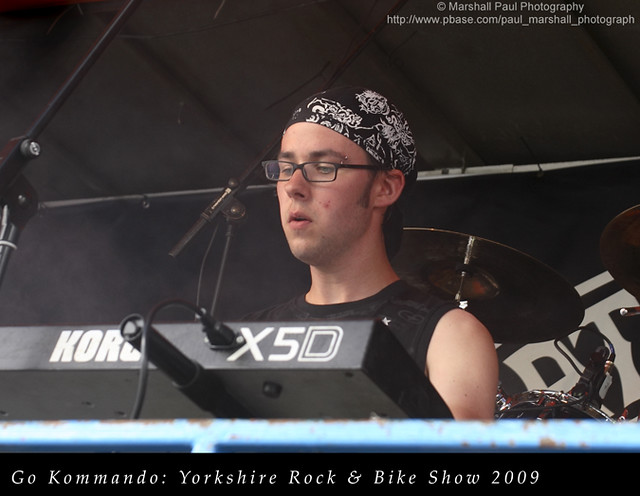The image captures a young man, likely in his early twenties, standing centrally in a landscape-oriented, color photograph. He is the focal point, positioned behind a Korg X5D synthesizer keyboard, with a microphone stand in front of him, indicating he might be performing at a music event. The setting appears to be either indoors or under a tent, reinforced by the enclosed ambiance. The young man dons a black and white bandana, black-rimmed glasses, and a black shirt, adding to the monochromatic theme prevalent throughout the image.

The background features a partially visible drum kit, further suggesting the musical context of the scene. Additional color touches include minor elements like rusty blue metal scrim. At the bottom of the image, a black banner stretches across, with white text that reads, "Go Commando: Yorkshire Rock and Bike Show 2009." In the upper right corner, another text segment credits the photographer, "Marshall Paul Photography," accompanied by the website "http://www.pbase.com/Paul_Marshall_photograph."

Overall, this detailed representation highlights the young musician engrossed in his performance, surrounded by his instruments and stage setup, with key textual elements adding context and credit.